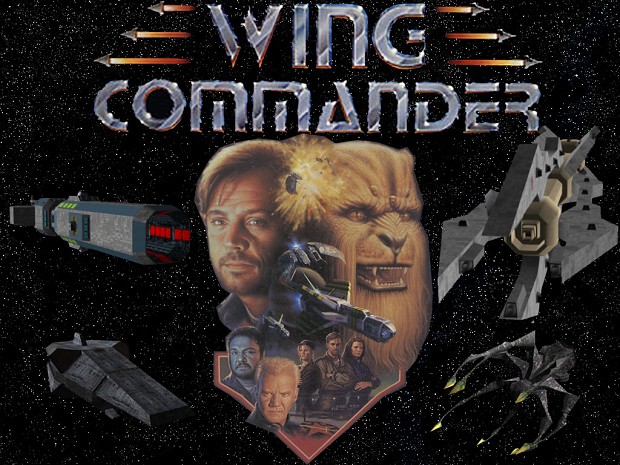The image depicts the cover art for the video game "Wing Commander," set against a black backdrop filled with numerous small white dots resembling stars. Central to the image is the title "Wing Commander," prominently displayed in a shiny, metallic silver font. Surrounding the title are six triangular spaceships, three on the left and three on the right, emitting orange-yellowish lines to signify firing lasers or propulsion.

Below the title, the central part showcases various characters from the game. Dominating the center is a male character with dirty orange-brown hair. Next to him is a lion-like creature with a golden mane and sharp teeth, reminiscent of a Chewbacca or Wookiee figure. Additional characters are distributed on either side: on the bottom left are two male figures, while the bottom right has three more characters. Accompanying these figures are several spacecraft, adding to the space-themed ambiance of the cover. The entire scene exudes a Star Wars-like feel, capturing an intense and adventurous outer space narrative.